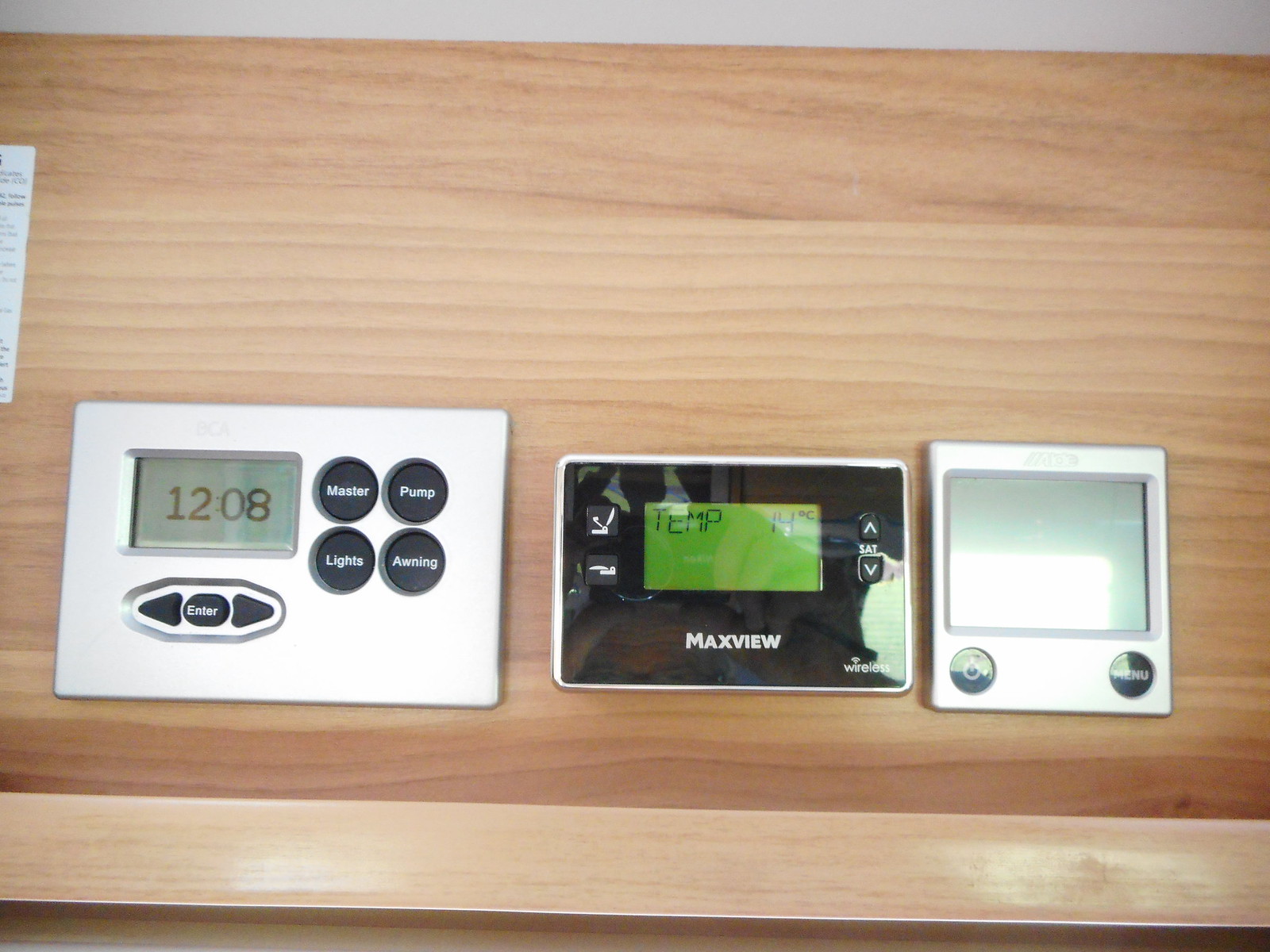The image showcases a row of three temperature control thermostats, aligned horizontally, mounted on a light brown wooden panel table. 

The leftmost thermostat is predominantly white and displays the time "12:08" in a black digital font set against a blue background. Below the time, there is an enter button shaped in an oval-rectangle hybrid with small arrows (carets) on each side, pointing left and right.

The central control unit has various circular buttons laid out in a grid. The top two buttons are labeled "Master" and "Pump," while the two below them are labeled "Lights" and "Awning." On the right, there is another button labeled "Max View." These buttons are all in white text against their respective backgrounds. Additionally, there is a button labeled "SAT" with white up and down arrows indicating adjustable settings.

The rightmost thermostat displays the temperature "14°C" on a green background. It features two additional buttons on the left. Unlike the first thermostat, this one does not show the time but includes a power button on the bottom left and a menu button on the bottom right, both in black circles with white text. This thermostat has a more square shape compared to the rectangular design of the one displaying the time.